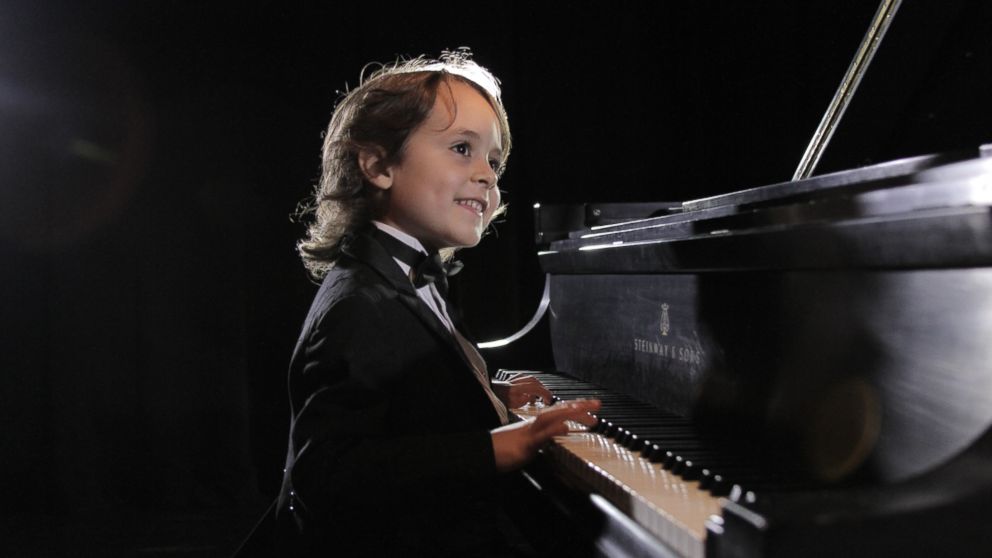In a staged indoor setting, a preteen boy with long hair extending past his shoulders is captured in a horizontally rectangular, full-color photograph. Dressed in a sharp black and white tuxedo with a clip-on bowtie, he is seated at a Steinway and Sons grand piano, identifiable by the distinct lettering and logo above the keys. The young pianist, who has a fair complexion and dark eyes, is smiling broadly as he looks toward his right, presumably at the audience. Both of his hands rest confidently on the piano's ivory keys. The scene is illuminated with artificial light, casting a gentle lens flare in the upper left corner and highlighting his hair. A silver pole, likely a microphone stand, is subtly visible beside the piano, blending into the dark black curtain backdrop.